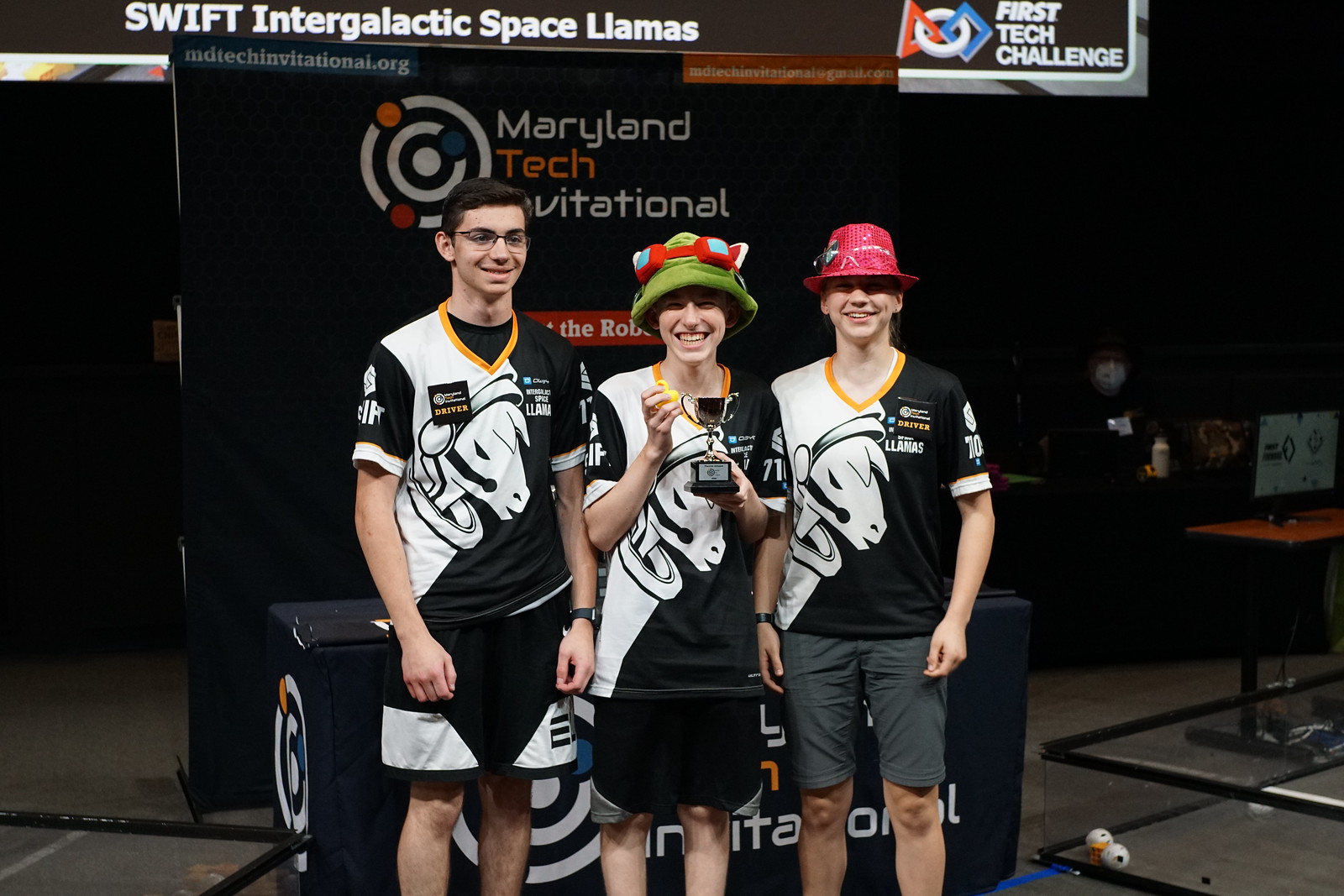Three young Caucasian students, dressed in similar uniforms featuring an image resembling a horse, stand proudly in front of a table covered with a black linen cloth displaying the same symbol as a poster behind them. The poster reads "Maryland Tech Invitational" and features a logo with orange, blue, and red circles forming a target-like design. The student in the middle holds a trophy, indicating their team has won some recognition in a tech challenge. Above them, a sign reads "Swift Intergalactic Space Llamas First Tech Challenge," likely the name of their team. Two of the students wear distinctive hats—one with a frog design and the other a red athletic cap. To the right, a short plexiglass box containing balls and a desk with a computer can be seen, while the overall background of the image appears dark, highlighting the participants and their accomplishment.